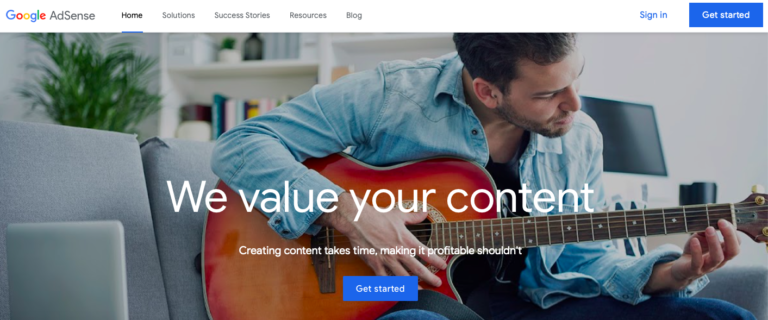The screenshot depicts a desktop view of the Google AdSense homepage. On the left side, the Google AdSense logo is prominently displayed alongside a navigation menu with tabs for Home, Solutions, Success Stories, Resources, and Blog. On the right side of the page, there are two buttons: "Sign In," which appears in blue text on a white background, and "Get Started," which is featured with white text on a blue background.

Below these buttons is a large, stock image of a man wearing a jean jacket, casually playing a nice guitar while sitting on a couch in what appears to be his home. The background includes a computer, some shelves, and a plant, lending a cozy, lived-in feel to the scene.

Overlaying the image is a prominent headline in white text that reads "We Value Your Content." Just below it, in smaller text, is the phrase "Creating Content Takes Time, Making It Profitable Shouldn't." Beneath this text, there is another "Get Started" button in blue.

The overall design of the page is clean and inviting, aimed at encouraging content creators to monetize their work through Google AdSense.